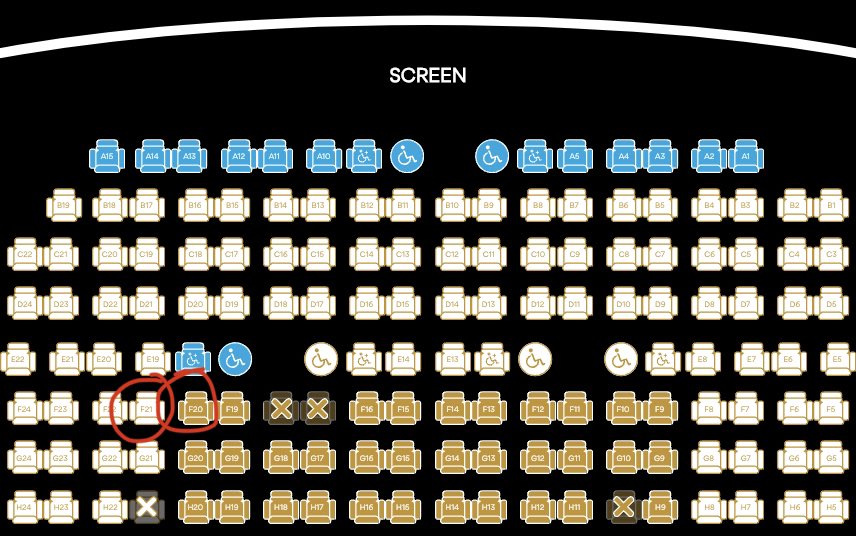This image is a screenshot depicting a detailed seating chart for an unidentified movie theater. Set against a black background, the chart features a prominent curved white line at the top labeled "Screen," indicating the location of the movie screen. Below the screen, multiple rows of seats are displayed in various colors, each representing different seating categories. The first row stands out in blue and includes two designated disabled seating areas. Subsequent rows are shown in white, with individual seats easily identifiable.

Notably, two specific seats near the back, labeled F20 and F21, are circled, drawing attention to their availability or special status. Additionally, some seats are crossed out, indicating they have already been reserved. These reserved seats are marked as F17, F18, H10, and H23. The chart does not provide information about the specific movie theater or the movie being shown. The image is strictly a graphical representation and does not include any photographic elements, people, animals, or botanical features.